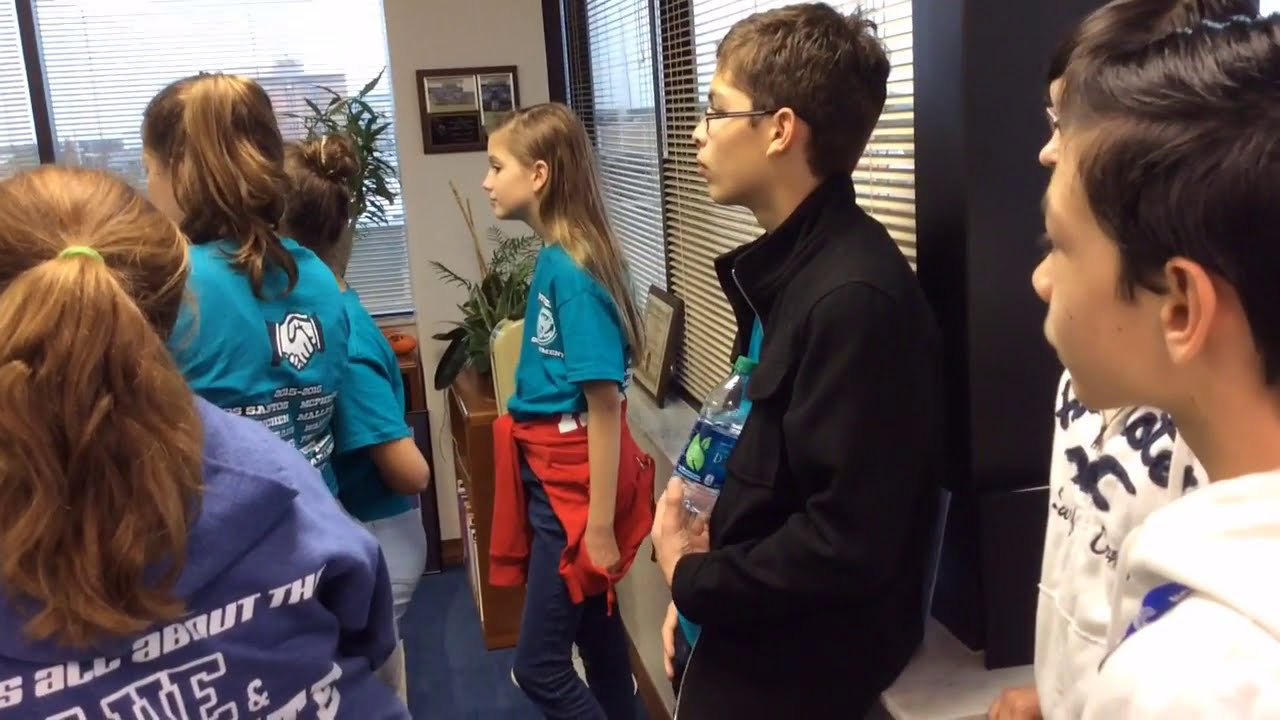The image depicts a group of children appearing to tour an office setting rather than a classroom. Positioned on the right side, several boys stand, each looking straight ahead. Notably, one boy with brown hair, wearing a black jacket, is centered slightly to the right, holding a water bottle. Behind these boys stand two males, both donning white hoodies with some wording on them, all looking in the same direction towards the left.

On the left side of the picture, there are several girls, predominantly with light brown or blonde hair. One girl in the foreground is wearing a turquoise shirt that features a handshake symbol on the back. Another girl, slightly farther back, is wearing a blue shirt.

The office interior is detailed with black-trimmed window frames that have white blinds, appearing to overlook a cityscape. The floor is covered in blue carpeting or tile. There is a small white pillar supporting a wooden plaque and a marble shelf beneath the windows against the back wall. Additionally, several potted plants and plaques are placed on a radiator and a table to the left of center. 

Overall, the children, a mixture of boys and girls, predominantly Caucasian, seem to be engaged in an organized meeting or tour within an office environment.